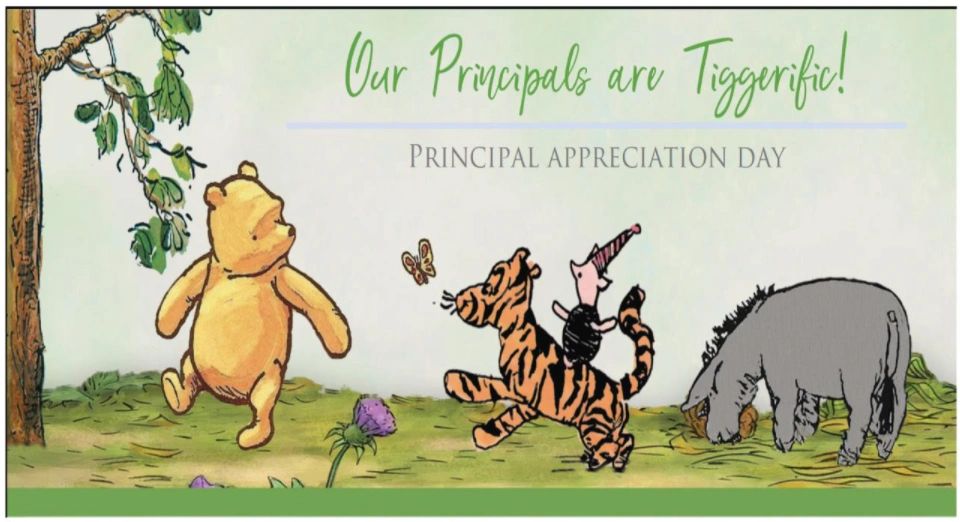This hand-drawn adaptation of the classic Winnie-the-Pooh characters serves as a whimsical poster for Principal Appreciation Day. The backdrop is a very light green, adorned with medium green script text reading "Our principles are Tiggerific." This text is accentuated by a light blue underline. Beneath this line, the phrase "Principal Appreciation Day" is inscribed in gray print. 

To the side, a hand-drawn tree boasts lush green leaves, rooted in a patch of green grass, with delicate purple flowers blooming in the foreground. 

In the center of this charming scene, Winnie-the-Pooh is depicted in mid-walk, glancing back at Tigger, who is joyfully chasing a yellow butterfly speckled with orange spots. Piglet, seated atop Tigger, sports a tall triangular hat and is donned in black clothing. 

To the side, Eeyore is munching on a bale of hay. His back is turned to the viewer, showcasing his tail and drooping ears, but not his face. This delightful illustration perfectly captures the playful essence of the Hundred Acre Wood gang, celebrating principals with a touch of nostalgia and affection.